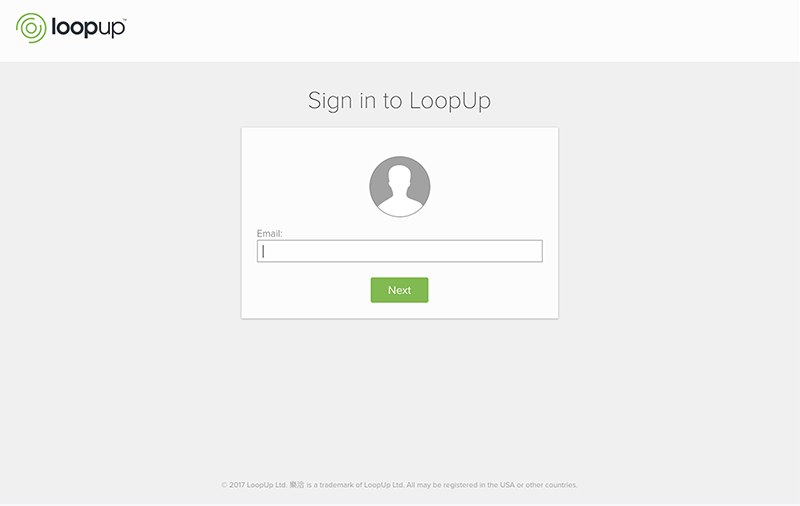The image features a primarily light gray background on the bottom part, spreading across the center and extending to the left and right sides. At the top portion, there is a thin, rectangular, horizontal box colored white.

In the top left corner of this rectangular box is a green logo, composed of partial circles that create a near-complete circle with segments missing; inside this main shape are smaller circles with a similar design.

Adjacent to this logo is the text "loop up," where "loop" is in bold black text and "up" is in standard black text.

Centered within the light gray area at the top, there is bold black text stating "Sign in to Loop Up," with the "L" and "U" in "Loop Up" capitalized. Below this text, a rectangular white box contains a light gray profile picture placeholder, depicting a simplified image of a person.

To the bottom left of the profile picture, "Email" is written in black text. Directly underneath this is a white entry field, outlined in light gray, suggesting an area where the user is expected to type.

Further down, there is a light green button with white text saying "Next." At the very bottom of the image, small, difficult-to-read light gray text appears. Starting from the left, it reads something akin to "2007 or 2017 Loop Up," with the remainder being too small and unclear to discern.